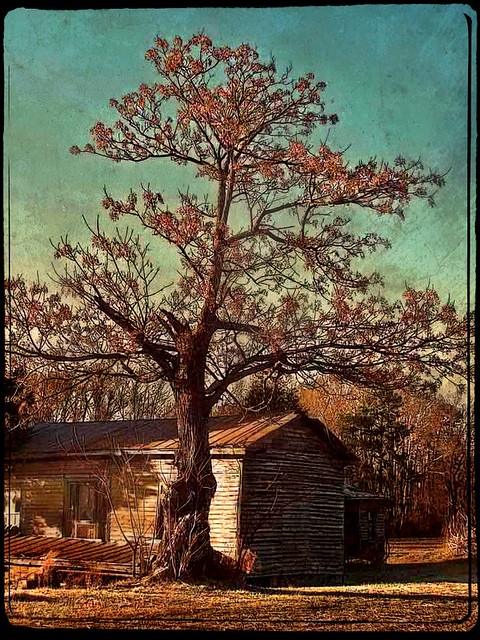The image depicts an oil painting of an old, rustic cabin or house situated in a relatively open woodland area. A large, twisted tree with reddish-orange, autumnal leaves towers above the cabin, its branches stretching across the scene and casting intricate shadows on the worn wooden structure. The sky is a vibrant blue with a clear, mottled appearance, adding to the serene yet slightly eerie atmosphere. The cabin, which features a rusted tin roof and chipping, peeling paint that once was white, shows signs of age and neglect, including moss growing on its left side and a window air conditioner unit framed with green wood. The ground in the foreground is scattered with fallen leaves, enhancing the autumn feel. Overall, the painting has a slightly washed-out, yellowish tint, suggesting that it has either been aged or the light during that time of day is creating a unique, faded effect.